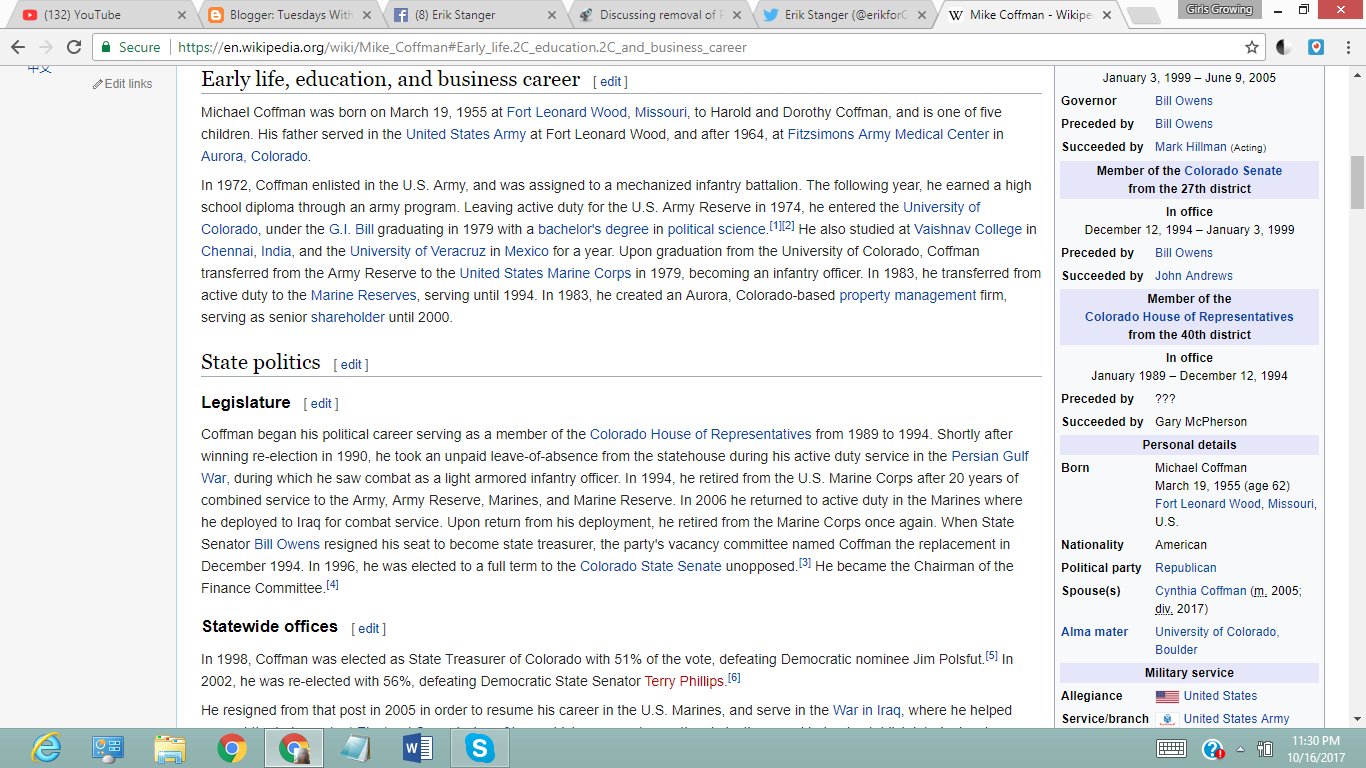This image shows a screenshot of a monitor displaying a Wikipedia page about Mike Kaufman. At the top of the screen, there are six open browser tabs. From left to right, they include:
1. A tab with the YouTube icon.
2. A Blogger tab with an orange icon featuring a white "B".
3. A Facebook tab labeled "Eric Stanger".
4. A partially visible tab with the text "Discussing Removal of".
5. Another tab labeled "Eric Stanger" with the Twitter icon.
6. A Wikipedia tab displaying "Mike Kaufman".

In the upper right-hand corner of the window, there's a red rectangle with a white "X" for closing the tab, and to its left, a gray icon labeled "Girls Growing". Below the navigation bar, the URL bar features a back arrow, reload button, and a blue secure padlock icon. To the right of the URL bar are a bookmark star and a split circle icon with black on the left and white on the right, followed by an additional blue icon.

On the webpage, the main headline reads "Early Life Education and Business Career" above the name Michael Kaufman. The page includes several paragraphs detailing Kaufman's early life. Following sections are titled "State Politics", "Legislature" and "Statewide Offices", detailing Kaufman's political career. Key information highlights his start in the Colorado House of Representatives and notes on his political career and achievements within the Colorado Senate. A vertical column on the right side of the webpage lists important dates and positions, including his term dates from January 3, 1999, to June 9, 2005, his role under Governor Bill Owens, and details about his succession in various roles. Additional details include his political party (Republican), spouse, alma mater, and other political allegiances.

Along the bottom of the screen, there is a blue-green toolbar that contains icons for various applications including:
1. Explorer
2. Monitor
3. File Manager
4. Google Chrome (two icons)
5. Notepad
6. Word processor
7. Skype

On the far right of the toolbar, a white typewriter icon and a blue circle with a white question mark are displayed. The timestamp at the bottom right corner reads 11:30 PM, 10.16.2017.